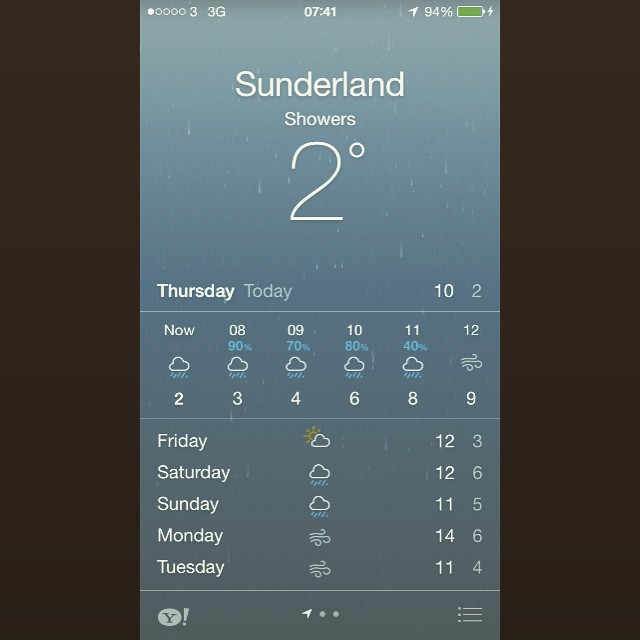Descriptive Caption:
The image depicts a screenshot from a weather application on a mobile device, likely a phone, given its rectangular shape with a taller-than-wide aspect ratio. The background is black, suggesting either a photo taken from a website or a pasted image. The weather app's interface shows a blue background at the top and includes status icons, such as a battery indicator, WiFi signal, and a 3G connectivity symbol. The time displayed is 7:41.

The weather information is for Sunderland, with a current condition of showers and a temperature of 2 degrees Celsius shown prominently. Below this, there's a calendar-like view presenting hourly weather updates for Thursday, starting from 8:00 AM to 12:00 PM. Each hour displays a rain cloud with corresponding rain probabilities: 90% at 8:00 AM, followed by similar predictions for the subsequent hours.

Further down, the app provides a five-day forecast from Friday to Tuesday. The first three days indicate rain, while Monday and Tuesday show windy conditions. Weather details for each day are organized into columns for dates, weather icons, and temperatures. Yahoo's logo at the bottom suggests that this weather app is powered by Yahoo.